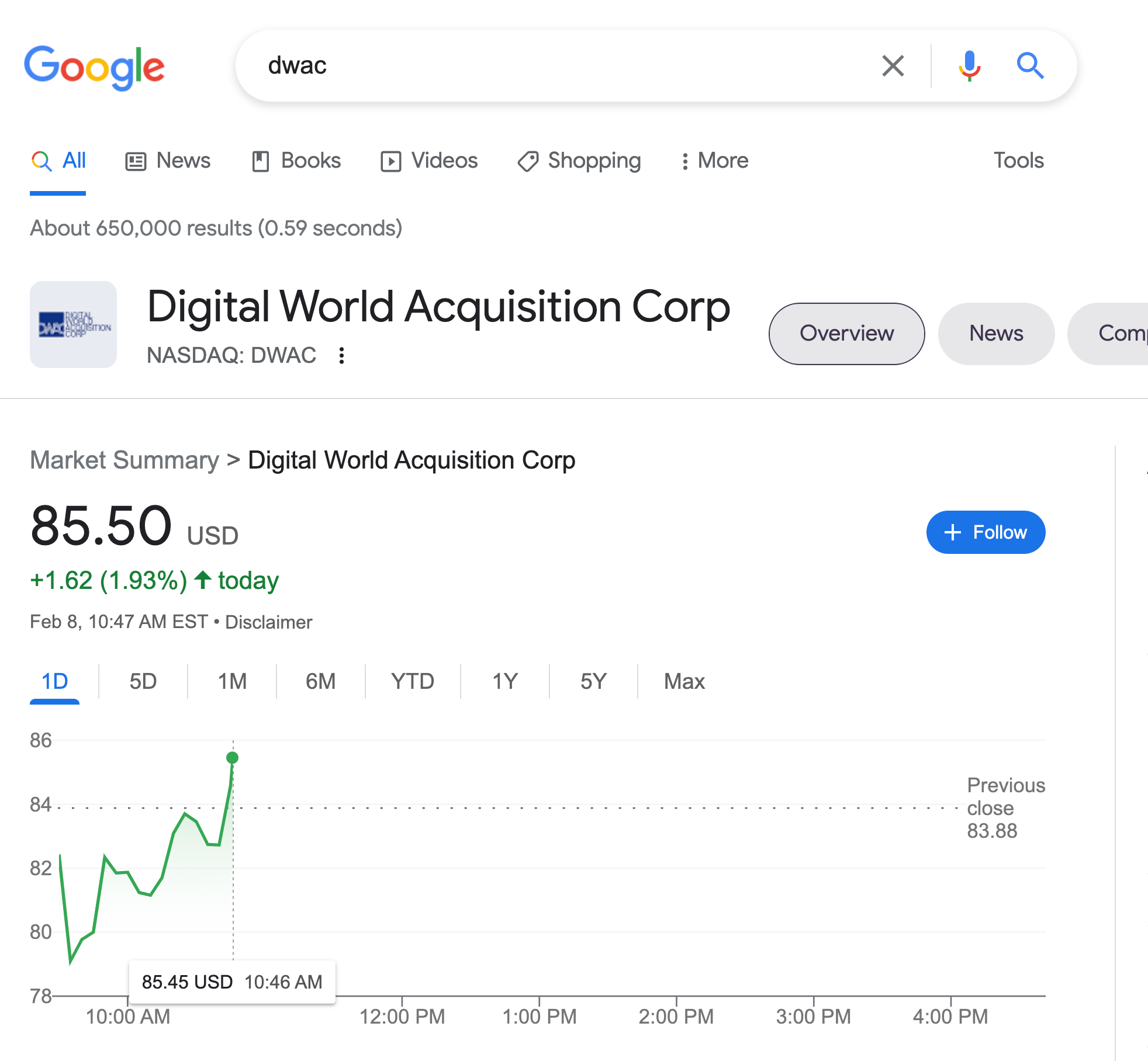Screenshot of a Google search results page displaying the stock performance of Digital World Acquisition Corp (DWAC). The multi-colored Google logo is situated at the top left, with the search bar to its right, containing the stock symbol "DWAC." Below the search bar, there is a navigation line offering options like All, News, Books, Videos, Shopping, More, and Tools, with the page showing approximately 650,000 results.

At the top of the results on the left side, there is a gray square area featuring the logo of Digital World Acquisition Corp. Next to this, the text "Digital World Acquisition Corp NASDAQ: DWAC" is displayed. To the right of this text are tabs labeled "Overview" and "News."

Beneath this section lies the market summary graph for Digital World Acquisition Corp. It is highlighted that the stock price is $85.50 per share, marking an increase of $1.62, or 1.93%, on this day. The date and time are recorded as February 8th, 10:47 AM Eastern Standard Time. The graph illustrates the stock's price movement over the past month, indicating an upward trend.